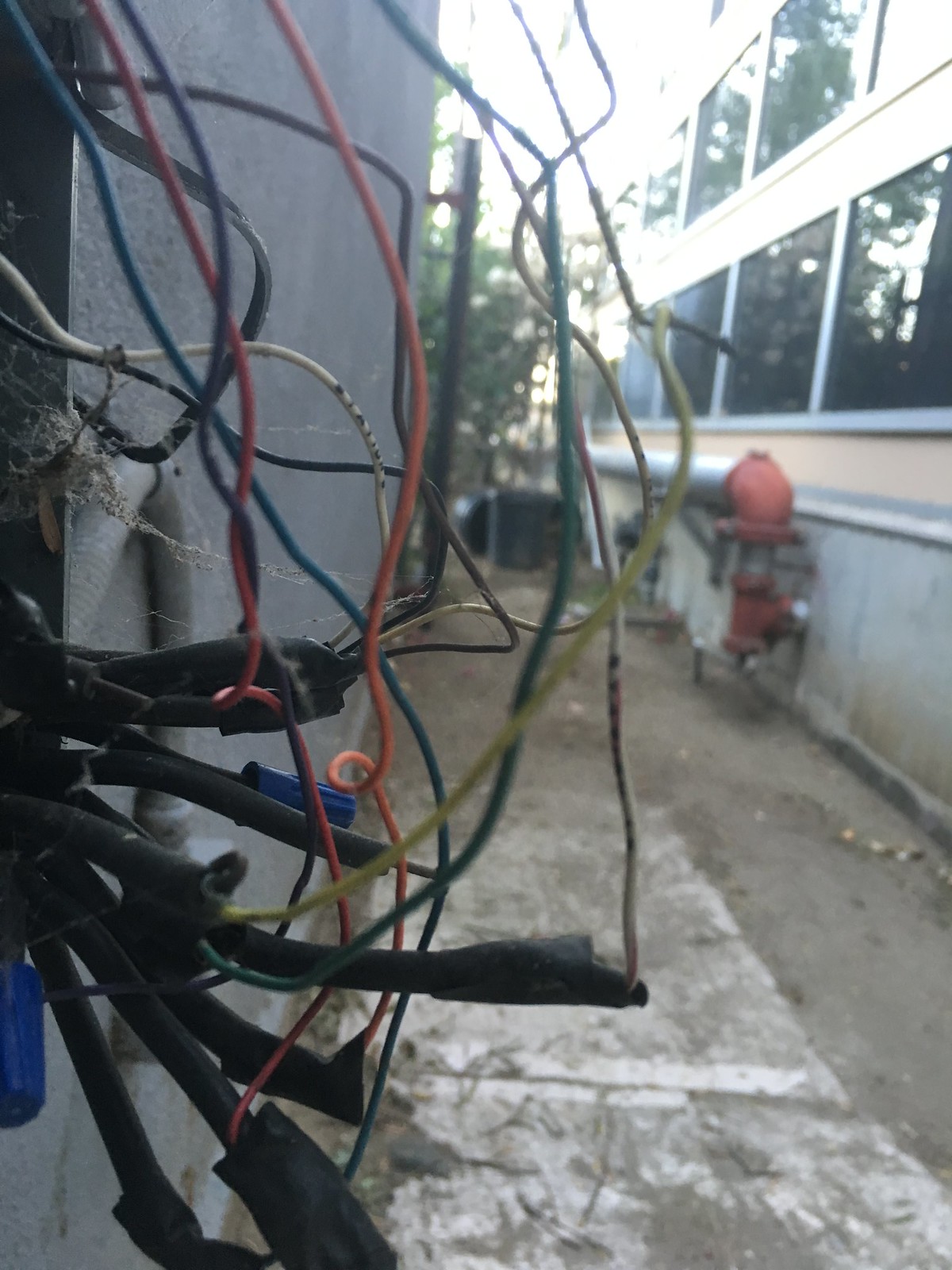The photograph depicts a chaotic cluster of colorful electrical wires emerging from a partially visible metal box mounted on a gray wall, possibly belonging to a home or business. The wires—yellow, blue, green, white, orange, red, black, and maroon—extend from the box and are bundled at their ends with black electrical tape or some kind of fabric wrap. A prominent spider web is tangled among the wires in the top left corner.

To the right of the image, a building with two tiers of long, reflective windows spans vertically. The building's exterior is color-blocked with a gray bottom, tan middle, and white top. A red, fire hydrant-like pipe runs along the side of the building, connecting to a larger gray cylindrical pipe.